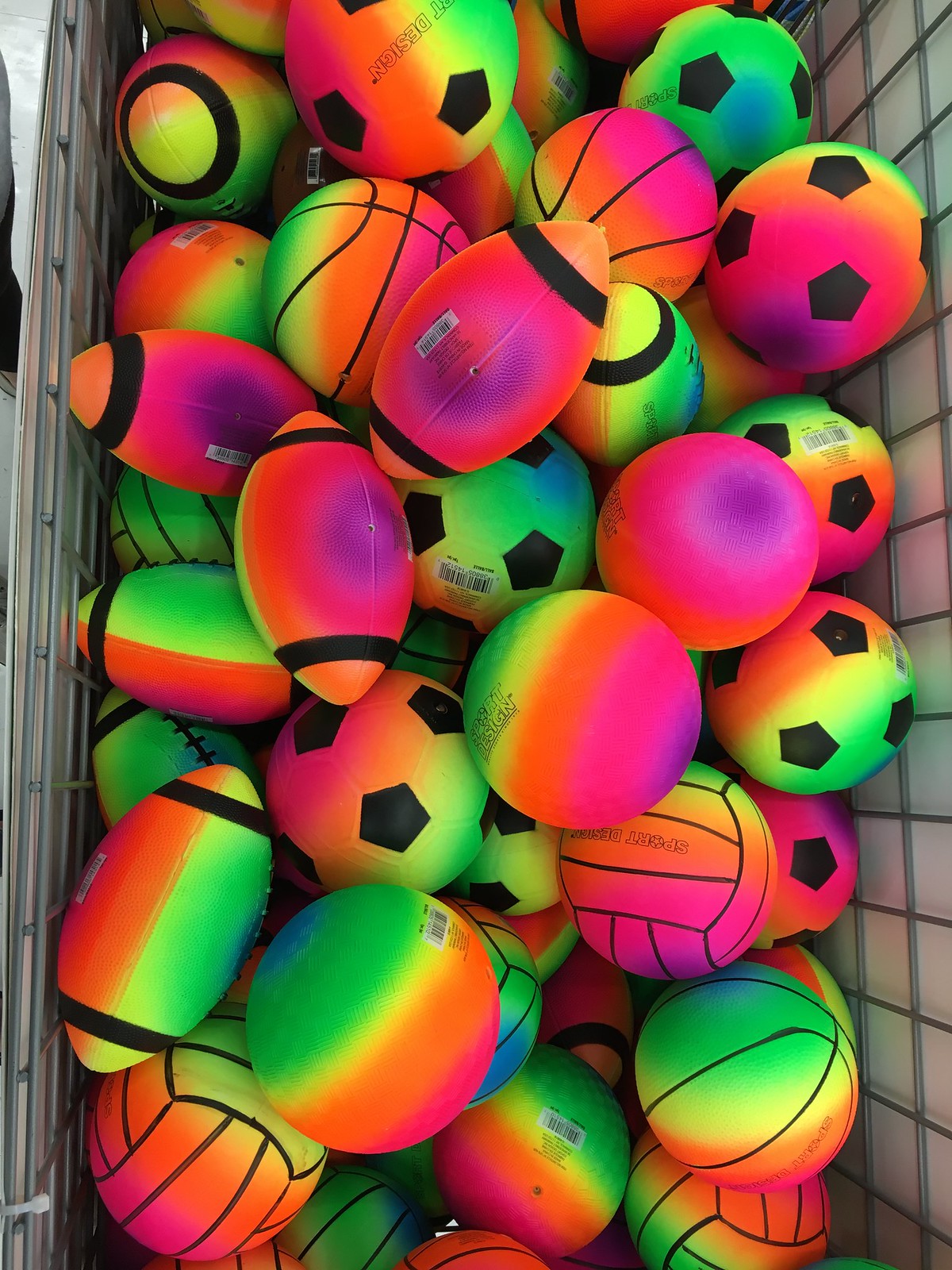The image captures a top-down view of a silver wire shopping cart or cage filled with various types of neon-colored sports balls. The balls include basketballs, soccer balls, footballs, volleyballs, and dodgeballs, all made from a Nerf-like foam material. Predominant colors are hot pink, bright orange, day-glow green, lemon-lime, yellow, purple, and blue, creating a vibrant pastel rainbow pattern. Each type of ball features distinctive black markings: soccer balls have black pentagons, footballs have black stripes at the ends, volleyballs have black stripes, and basketballs are marked with black piping. Some balls bear small writing and UPC symbols. The cage contains around 30 to 40 balls, all piled together in a colorful and orderly manner.